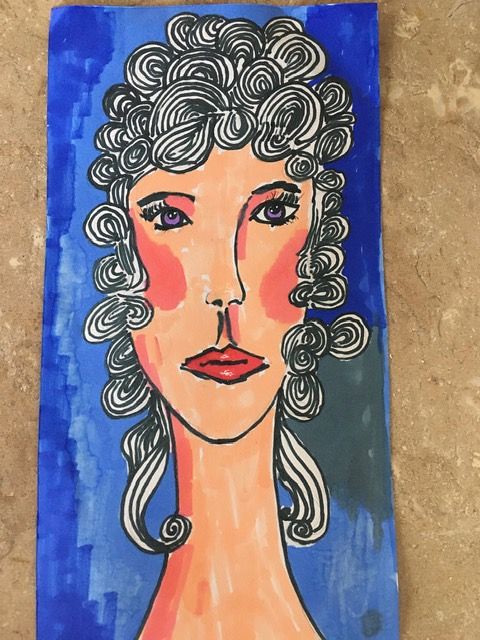This image portrays a detailed illustration that appears to be a painting, laid flat on what seems to be a table. The painting features a background imbued with a watercolor-like effect in various shades of blue, interspersed with hints of black, giving it a depth and fluidity. Central to the piece is the depiction of a woman with a strikingly elongated neck and face. Her eyes, a mesmerizing bluish-gray, are accentuated with long, delicate lashes. Rosy cheeks provide a touch of warmth to her face, which further elongates along her nose. Her lips are painted a vibrant red. The woman’s hair, a mix of black and white, is styled in distinct, vintage curls that fall just below her chin, adding to the timeless elegance of the artwork.